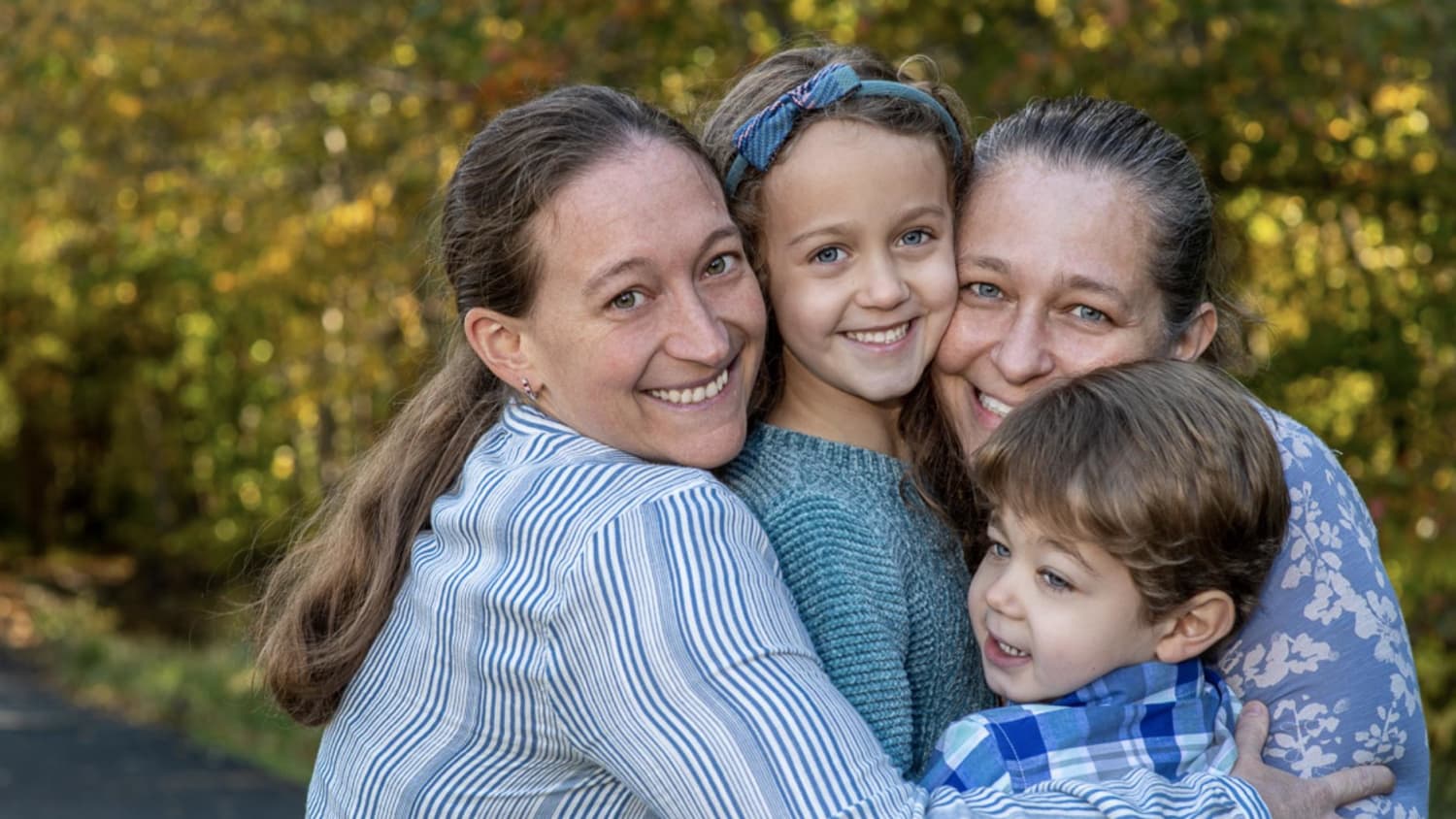In this photograph, we see a loving family embrace amidst a picturesque outdoor setting. The background features a blurred line of trees, with shades of yellow and green, and sunlight streaming through, casting a warm glow on the dark gray or black road. Centered in the frame are two women and two children, all displaying joyful expressions. 

On the left stands a middle-aged woman with long brown hair tied in a ponytail, lighter at the ends than near her crown. Her blue shirt with white stripes adds to the harmonious color palette. Beside her is a young girl, around eight or nine years old, with brown hair adorned with a blue bow featuring purple and blue stripes. She mirrors the woman’s smile and wears a teal sweatshirt that complements her striking blue eyes.

Lower down, a young boy, probably four or five, with short brown hair looks away towards the left. His outfit—a plaid shirt in various shades of blue and white—matches the family's blue-themed attire. 

On the right is an older woman, likely the grandmother, as suggested by her gray hair and the familial resemblance she shares with the woman on the left. She, too, has blue eyes and is smiling, although the boy's head slightly obscures the right side of her face. Her blue and white floral dress enhances the tranquil and unified appearance of the group. The women, with their similar features and hairstyles, could be twins or mother and daughter, adding a layer of generational beauty to the photo.

All four individuals are tightly hugging one another, radiating warmth and affection, captured perfectly in this heartfelt family moment.